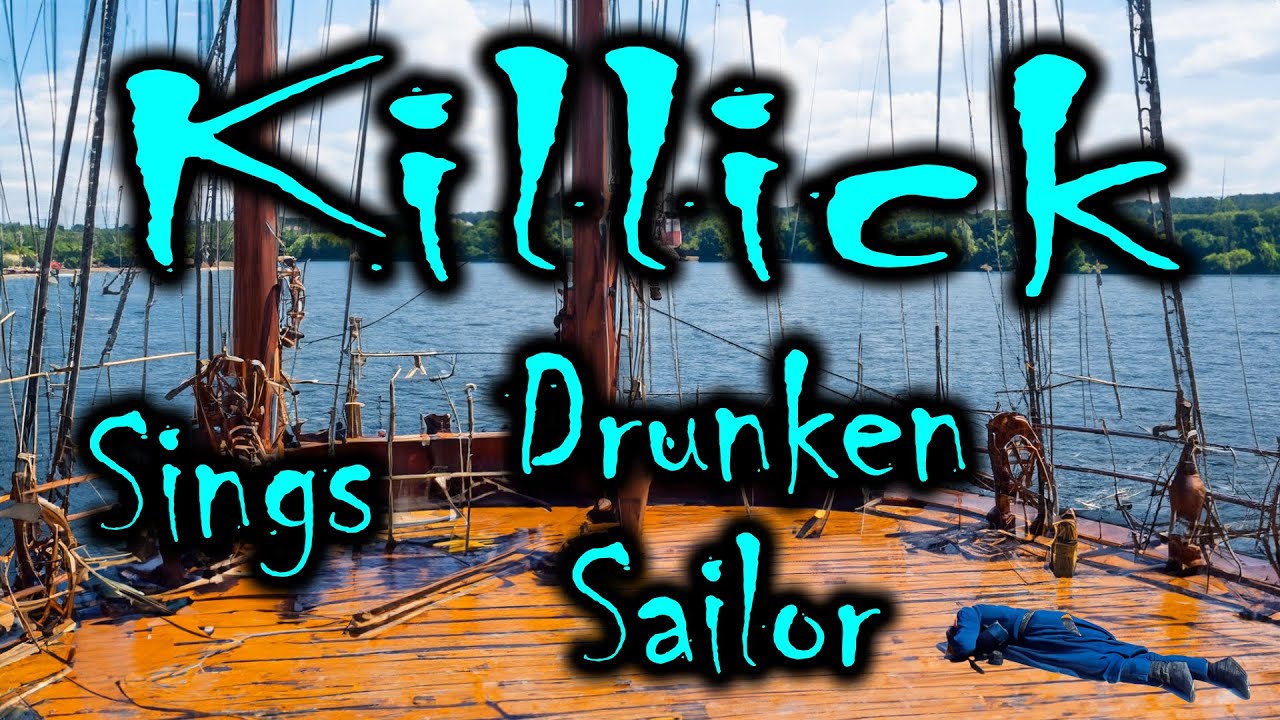The image depicts a scenic photograph of an old sailship with a weather-worn wooden deck. In the foreground lies a person dressed entirely in blue, including blue pants, shirt, and black boots, sprawled face down on the deck. This person's head is not visible, adding an element of mystery to their state, possibly suggesting they are the "drunken sailor" referred to in the text across the image. The ship floats on a vast body of blue water, with a lush, green forest and small houses faintly visible along the horizon under a partly cloudy sky. Adding a contrasting and somewhat cheesy element, bold teal graffiti-style text stretches across the photograph, reading "Killick Sings Drunken Sailor," which might indicate a promotional poster for a band or a themed event. The juxtaposition between the serene backdrop and the informal text creates a unique, if slightly incongruous, visual experience.